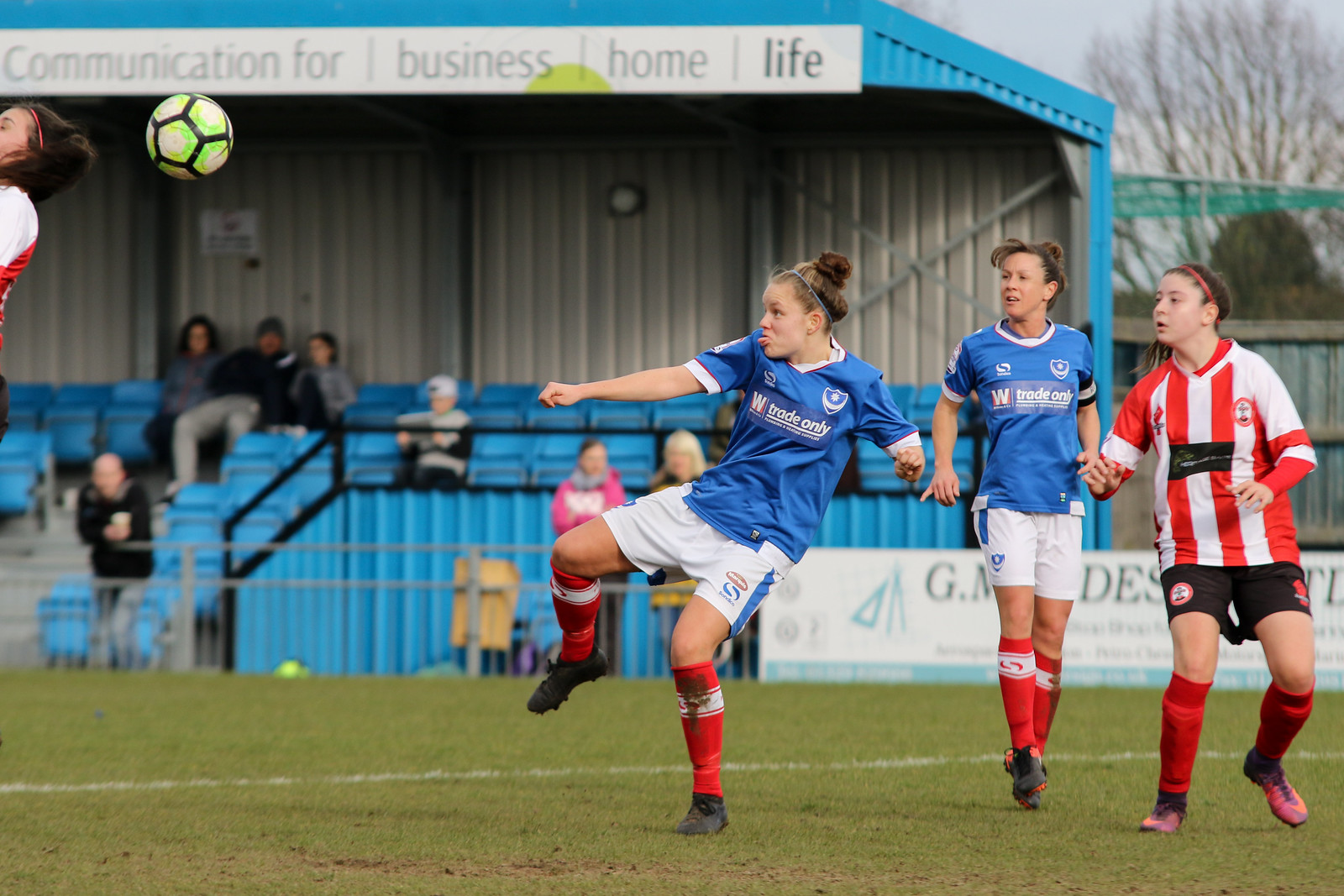In the photograph, a group of female soccer players are captured in an intense moment on the field. Two players wear blue and white soccer uniforms paired with red socks, while a third player dons a red and white jersey with black shorts and red socks. The action centers around a green and black soccer ball that one of the blue-uniformed girls has just kicked, sending it airborne. The scene is set against a backdrop of blue and black bleachers, where a few spectators, including two middle-aged women, watch the game unfold. A sign atop the bleachers reads "Communication for Business, Home, and Life," indicating a sponsor. The player in the center, who appears focused with her tongue slightly out, seems either to have just kicked the ball or is preparing to receive it. Despite the overcast daylight, the energy of the moment is palpable.